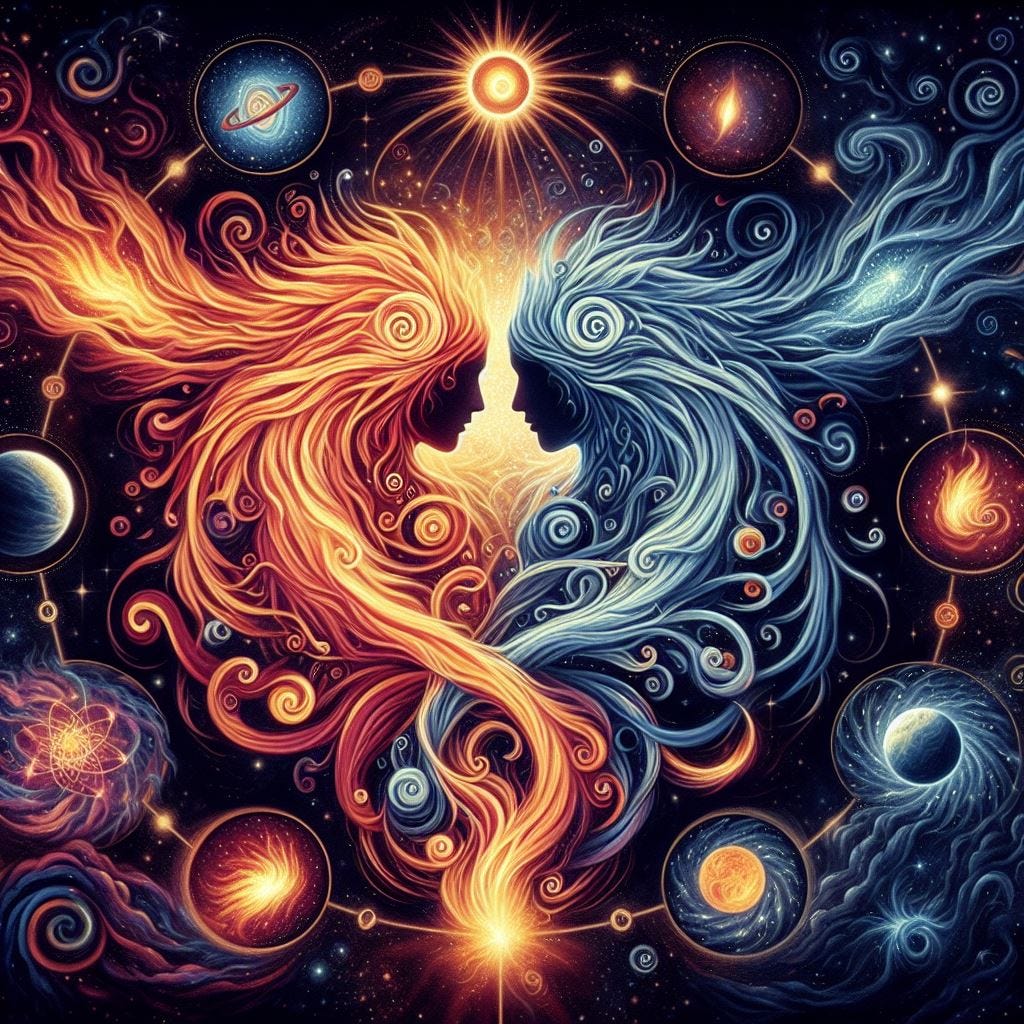This square-shaped digital artwork features two feminine silhouettes facing each other against a dark night sky. Their heads are slightly bowed, with bright white light emanating from behind them. The woman on the left has flowing, fiery hair in varying shades of gold and orange, while the woman on the right has silver-blue hair reminiscent of ice. Their hair swirls and intertwines towards the bottom center of the image. Surrounding these central figures is a circular gold ring adorned with nine circles, each depicting different celestial objects or nebulas. The outer corners of the piece are embellished with loose, swirling nebulous designs, enhancing the fantastical, space-themed ambiance of the artwork.